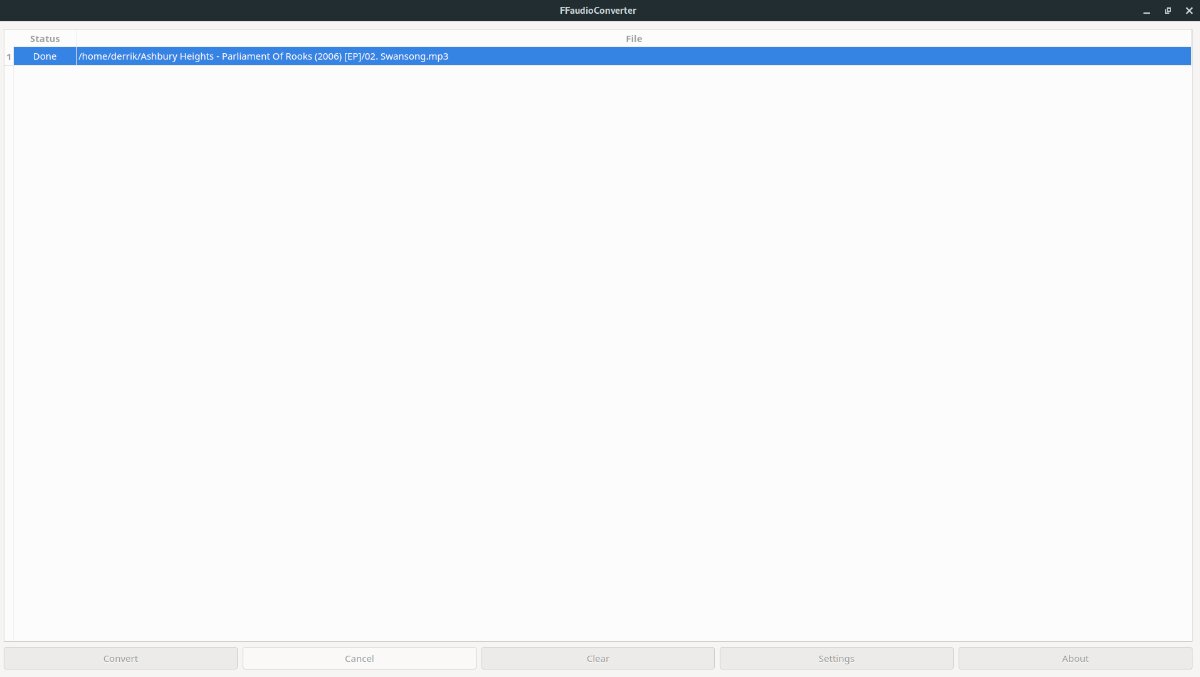This detailed screenshot captures a tab within a converter application, made more visible due to cropping and enlargement, albeit causing slight blurriness in text.

At the very top, a black header carries the app title centrally positioned, displaying "FF [Word] Converter" in a small white font. Below this, the main body of the application bears a white background. In the upper left corner, "Statuses" is inscribed in extremely tiny gray print, mirrored by the word "File" in equally minute gray print in the center.

Subsequently, under the "Status" label, the term "Done" indicates a completed task, adjacent to which stands the file name ending in ".mp3" on the right.

The remaining expanse of the page stays blank, leading down to the bottom of the application where five vertically aligned gray buttons are displayed: "Convert," "Cancel," "Clear," "Settings," and "About." Notably, the "Cancel" button is highlighted in white, indicating it has been selected.